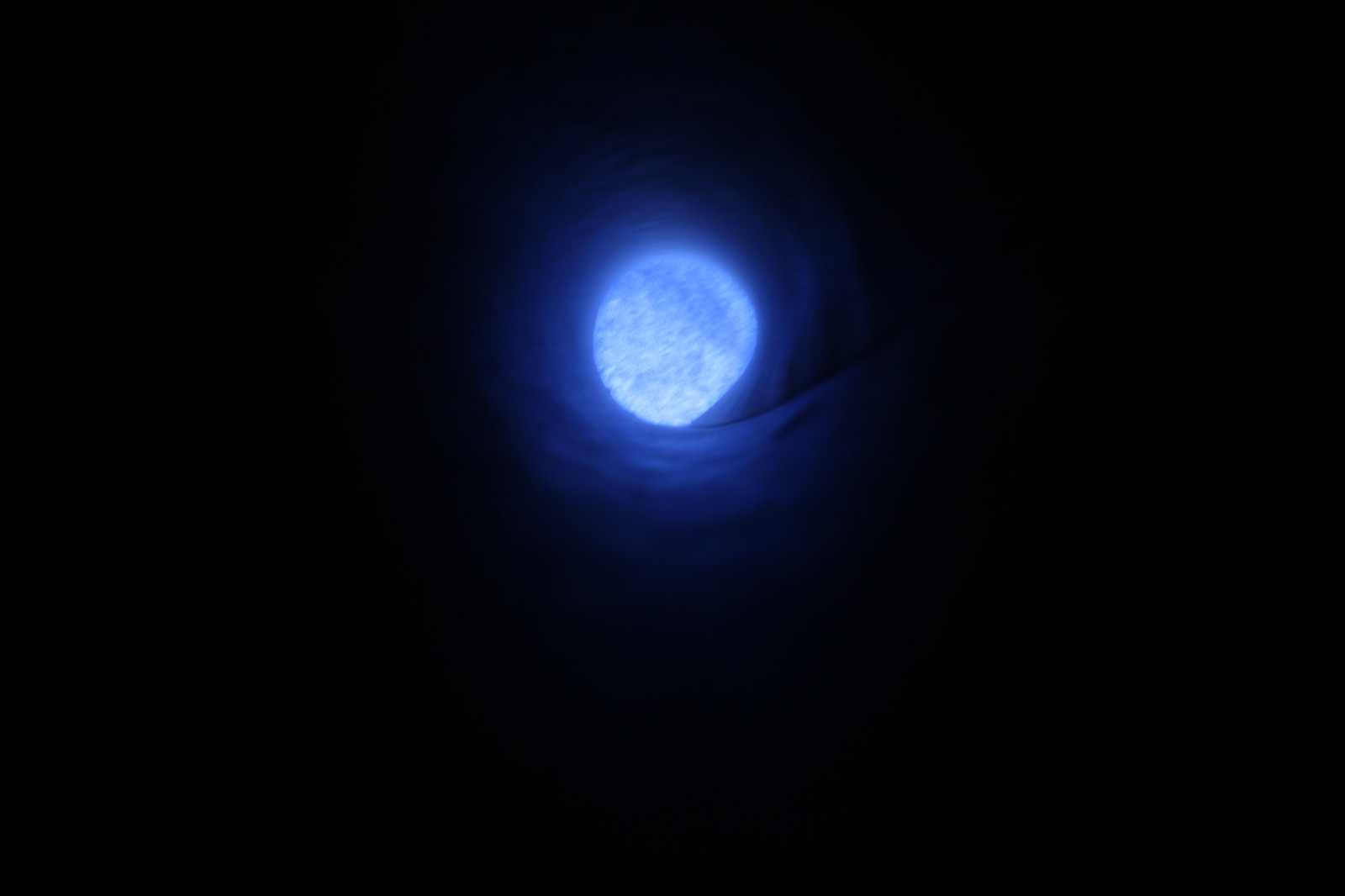The photograph is a striking night-time image featuring the moon at its center. The background is a jet-black sky devoid of any stars, which accentuates the central focus on the moon. Encircling the moon is an eerie, luminous blue glow that has a shadowy or smoky quality, likely caused by illuminated clouds. This glow enhances the mysterious ambiance of the scene. The moon itself is a haunting grayish-blue, with darker gray markings that reveal its craters and surface details. Interestingly, the perspective could be interpreted as looking up through a circular tunnel or a telescope, giving the impression of the moon’s light illuminating the edges of a rounded structure. Adding an enigmatic touch, a single red dot is visible above the moon, possibly indicating a distant star or another celestial object, further enriching the captivating and otherworldly quality of the image.